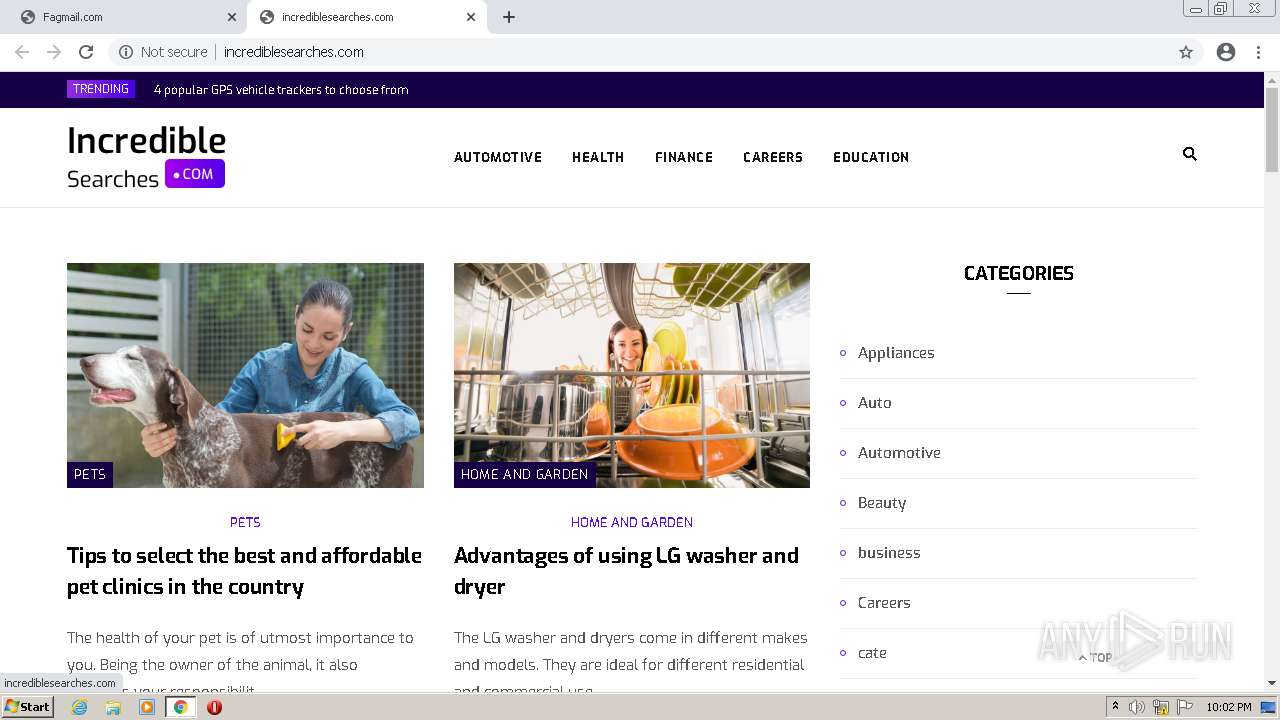This is a screenshot of a webpage displayed on an old Windows Vista operating system. At the top of the screenshot, the browser is opened with two visible tabs. The active tab shows the website "incrediblesearches.com" in the URL bar. Below the URL bar, a purple banner with slightly blurry text displays "Trending: Popular GPS Vehicle Trackers to Choose From." On the left side of the banner, the website's logo, "incrediblesearches.com," is prominently displayed. To the right, the navigation menu includes categories such as Automotive, Health, Finance, Careers, and Education.

The website itself has a clean, white background featuring various articles. Each article is accompanied by a category image, followed by descriptive headlines. At the bottom of the screenshot, the familiar old Windows Vista taskbar is visible, adding a nostalgic touch to the overall image.